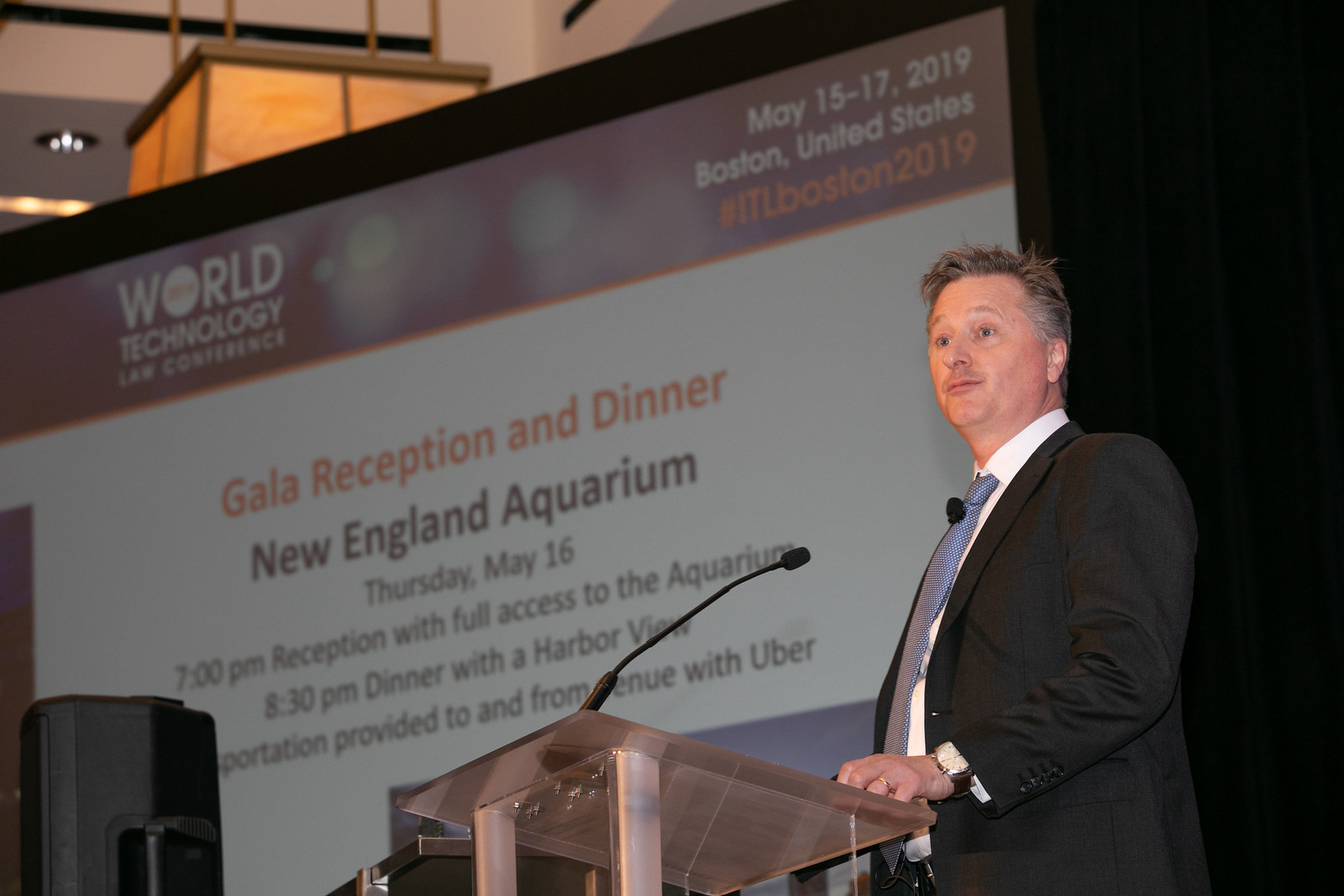This horizontally aligned rectangular image captures a man in his 40s standing at a silver podium with a thin attached microphone, speaking at an event. He is a white male with short gray and brown hair, dressed in a black suit jacket, white collared button-down shirt, and a blue tie. He wears a watch and a ring, and his hands rest on the podium. Behind him is a large projected screen with the heading "World Technology Law Conference" in the upper left-hand side and the event details "May 15 through 17, 2019, Boston, United States" in the upper right-hand side. The center of the screen announces the "Gala Reception and Dinner" at the New England Aquarium on Thursday, May 16, with a 7 p.m. reception granting full access to the aquarium and an 8:30 p.m. dinner with a harbor view. It also notes that transportation to and from the venue is provided via Uber. The backdrop of the scene includes long black curtains and some visible overhead lights, creating an indoor presentation hall atmosphere. The man appears to be addressing a question from the audience, emphasizing his engagement with the attendees.